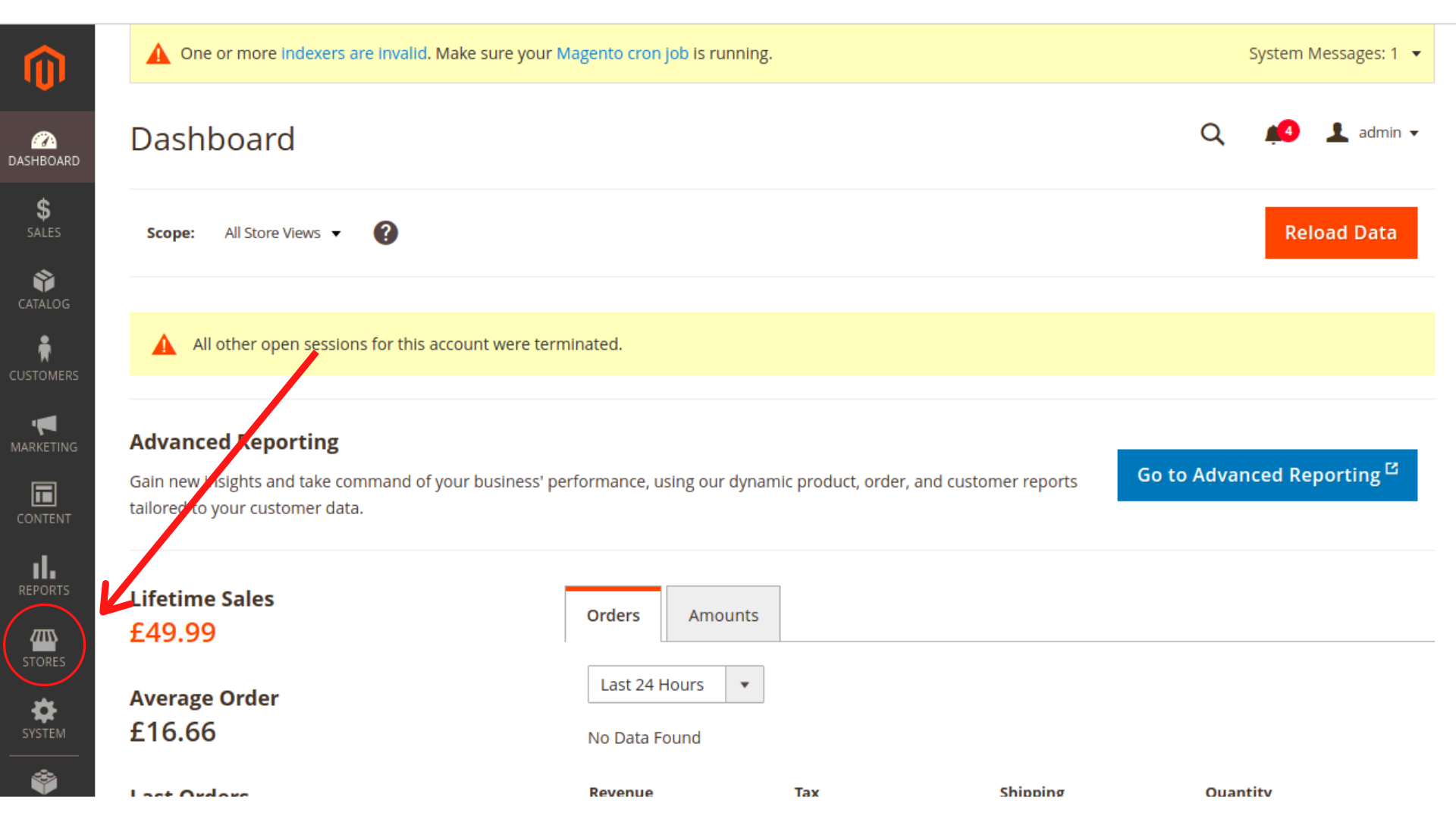This image showcases a dashboard interface, possibly for an e-commerce platform like Magento. The layout is meticulously structured for ease of navigation and functionality. 

**Left Column:**
- The left sidebar is black and displays an orange logo at the top, consisting of two 'U's, one smaller and one larger, possibly a stylized representation of the platform's branding.
- The sidebar elements include:
  - **Dashboard:** (Highlighted)
  - **Sales**
  - **Catalog**
  - **Customers**
  - **Marketing**
  - **Content**
  - **Reports**
  - **Stores:** (Circled with an arrow pointing to it)

**Body of the Page:**
- At the very top, a system message declares, "All other open sessions for this account were terminated."
- A warning triangle icon is accompanied by a notice, "Indexes are invalid. Make sure your Magento cron job is running."
- To the right of this notice are system messages with a dropdown arrow for additional options.
- Below the system messages, the word "Dashboard" is prominently displayed in white.
- To the right, a set of icons and functionalities are arranged:
  - **Search** icon
  - **Notification** icon with four notifications
  - **Admin** section with a dropdown arrow
  - **Scope:** Displaying "All Stores" with a dropdown arrow
  - **Question** icon
  - **Reload Data**

**Main Content Area:**
- Below the highlighted attention triangle and the repeated session termination notice, there is a section for advanced reporting. It reads, "Gain new insights to take command of your business performance using our dynamic product order and customer reports tailored to your customer data."
- A blue button labeled "Go to Advanced Reporting" is positioned to the right.
- Further down, there is a financial summary:
  - **Lifetime Sales:** €49.99
  - **Average Order:** €16.66
- Two tabs, one for "Orders" (highlighted) and another for "Amounts," are displayed.
- A dropdown box allows selection for the time frame of the data, currently set to "Last 24 hours."
- Below this, various metrics labeled as "Revenue," "Revenue Tax," "Shipping," and "Quantity" are noted, though no data is found.

Overall, the dashboard uses clear sectioning and annotations to ensure the user can efficiently manage and analyze business operations.